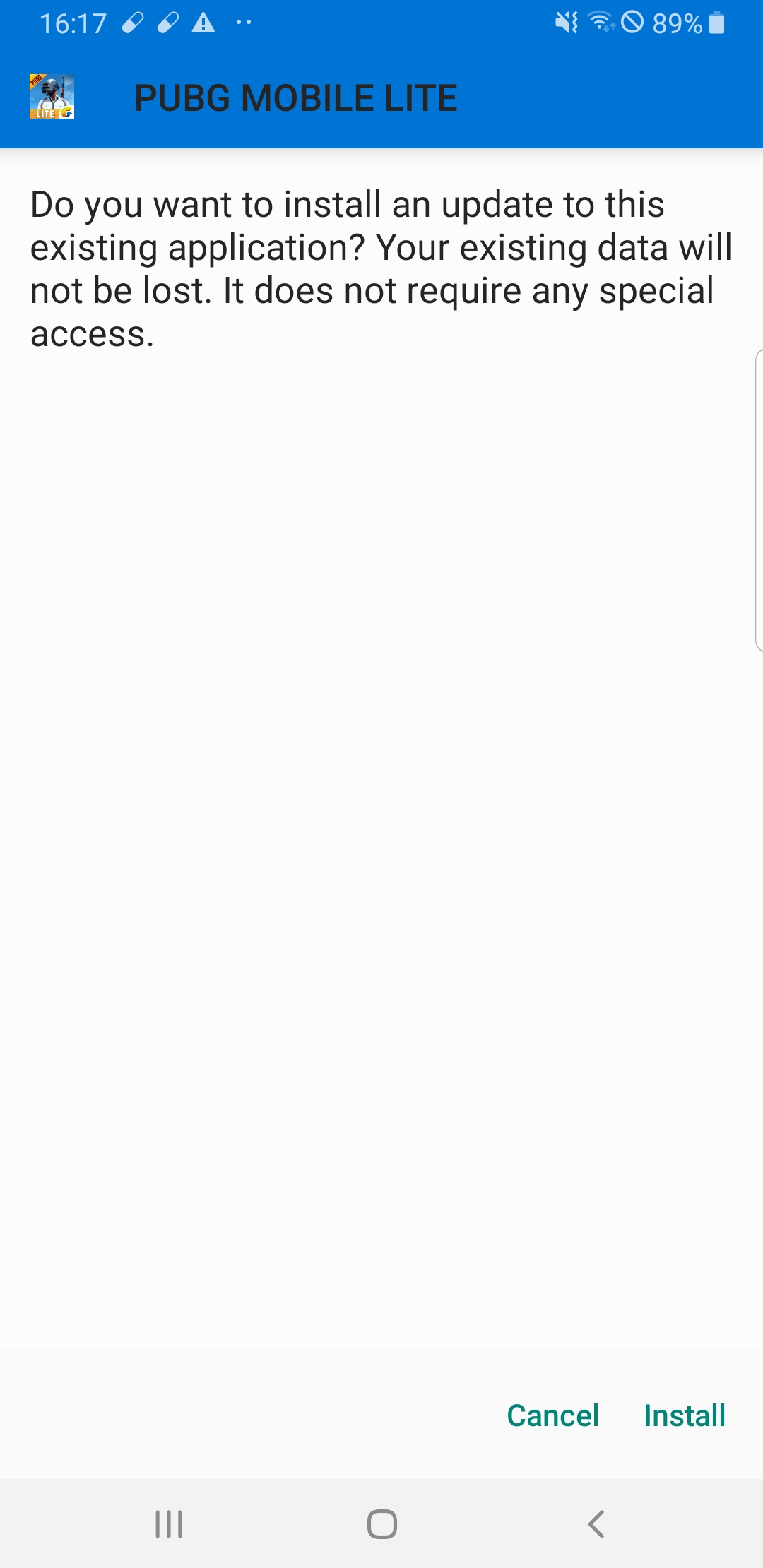A close-up image of a smartphone screen displaying an update prompt for the "PUBG Mobile Lite" application. The screen message reads: "Do you want to install an update for this existing application? Existing data will not be lost. Does not require any special access." At the top of the screen, there's a small icon featuring a character in a helmet, representative of the game's logo. The background of the prompt is predominantly white, with blue accents at the top. The options to "Install" or "Cancel" the update are prominently displayed at the bottom in green buttons. The interface is simple and uncluttered, indicating an easily navigable update process. This is typical behavior for app updates, aiming to ensure all users have the latest features and fixes.